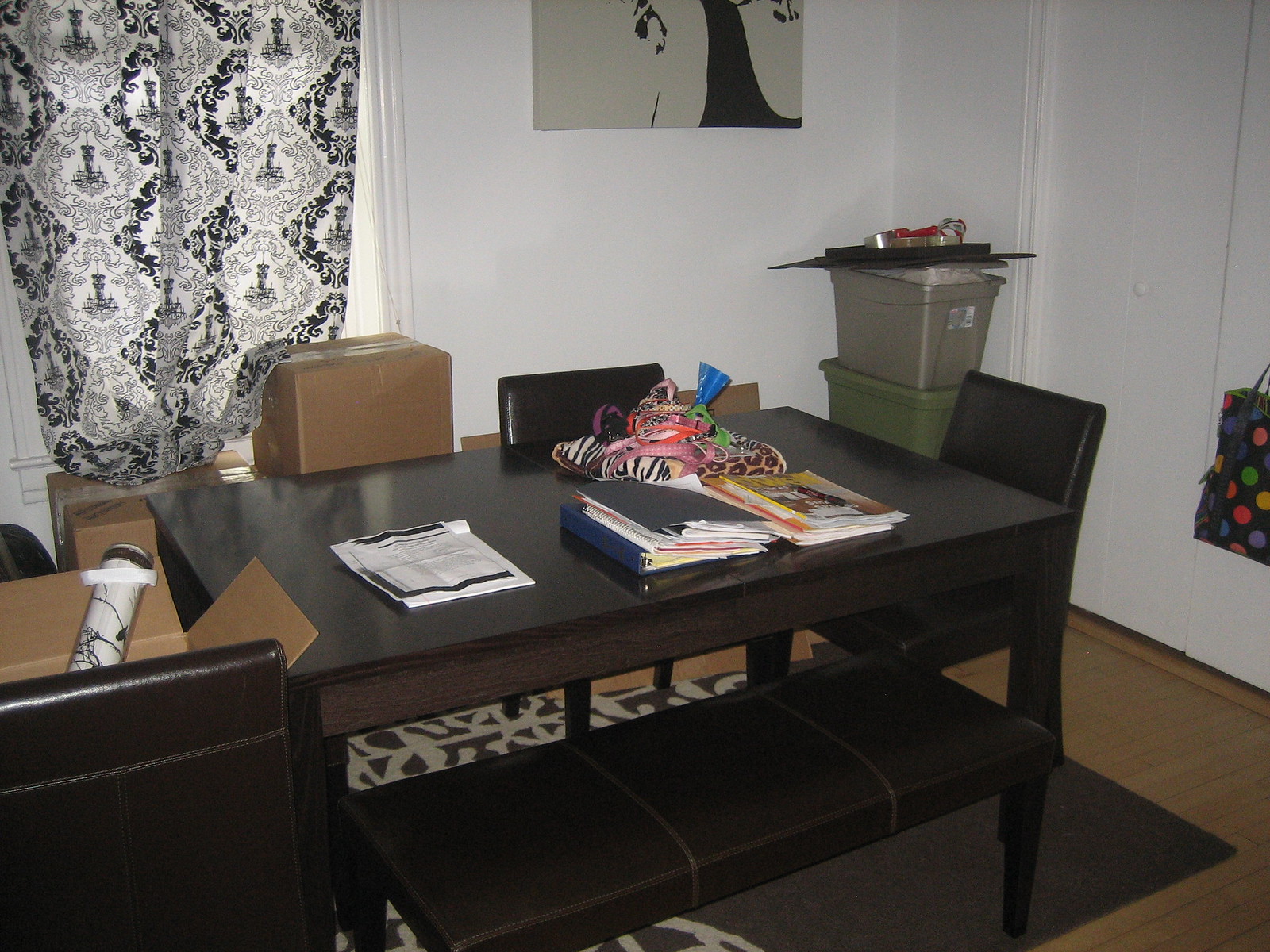This detailed, horizontal rectangular photograph captures the interior of what appears to be a cozy den within a home. Central to the scene is a dark chocolate brown wooden table, positioned diagonally towards the lower right corner. Accompanying the table are two dark brown or black leather chairs; one chair's back is facing the lower right corner, while the second chair gives a partial view of its back and seat cushion facing the right edge. The table surface is cluttered with a variety of items: a stack of notebooks and folders with papers protruding, similarly sized softback books nearby, a collection of different colored items behind the notebooks, and loose papers to their left.

In the background, to the left of center, sits a sealed cardboard box, positioned near or against the table. A black and white curtain adorns a window, their accompanying white trim descending from the upper left corner to the mid-level of the photograph. The top portion of a canvas painting, depicting a gray background with a black tree trunk, decorates the wall.

The right side of the image features white closets with matching white knobs, extending three-quarters down to intersect slightly towards the middle. A colorful, circle-patterned bag is partially visible, hanging by its strap near the closet. Additionally, two large, olive green Tupperware boxes are stacked a little right of center, roughly a third down from the top. The top box has a white label facing outward and is topped with miscellaneous items.

The floor showcases a medium brown wooden finish with visible planks, complemented by a chocolate brown area rug with a white pattern. Situated in the left-hand corner is an opened cardboard box, one flap leaning against the table, revealing a poster tube in white and black inside.